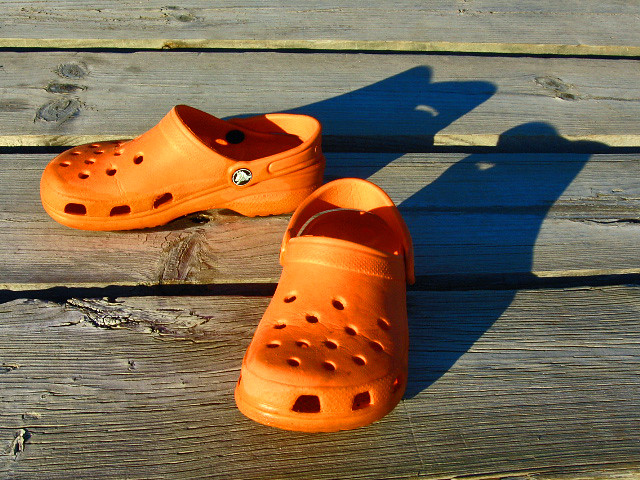In this detailed photograph, a pair of orange Crocs are prominently featured, resting on a weathered wooden deck composed of light-colored, horizontally-laid planks. The top plank extends beyond the top edge of the image, while the following three planks run towards the viewer in perspective. The third plank is slightly cropped at the bottom. The Crocs exhibit distinctive features including ventilation holes at the top and sides and are crafted from a soft, rubbery material. One shoe, located near the bottom center of the image, faces the viewer, while the other shoe, positioned higher up and to the left, lies perpendicular to its pair, showcasing a round black insignia. The deck wood is marked with natural striations, knots, and notches, and is illuminated by a bright light source from the lower left, casting sharp shadows behind the shoes to the right. This combination of elements creates an artistic and visually engaging composition.